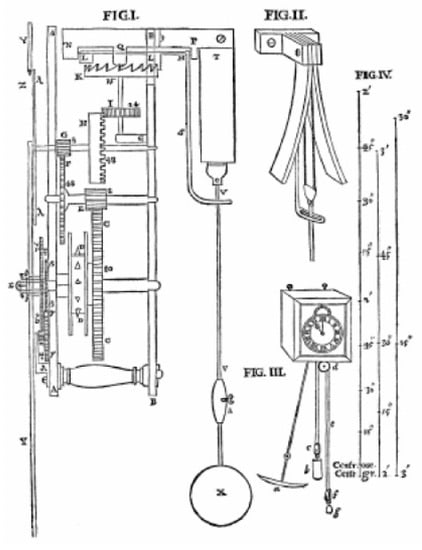The image is a detailed black-and-white schematic drawing, divided into four distinct figures labeled with Roman numerals I through IV, presumably illustrating different components of a clock mechanism.

**Figure I:** This section presents a mechanical construction featuring various interlocking gears, switches, and rods. At the lower part of this figure, a string or wire and a large round weight or pendulum base can be seen, hinting at its function within a pendulum mechanism. The interconnected parts suggest a complex motion system that may drive the clock's internal operations.

**Figure II:** Positioned towards the top-right of the image, this figure depicts a T-shaped contraption, identifiable by a handle and an overhanging flap or pendulum-like extension. This structure appears to resemble a metronome-like system or another mechanical component contributing to the clock's regulation.

**Figure III:** Just below Figure II, this part of the diagram centers around a clock face enclosed within a rectangular boundary. Directly beneath the clock face, there's a swinging device, again possibly a pendulum, essential for maintaining accurate time through its rhythmic motion.

**Figure IV:** Located on the far right of the schematic, this figure appears to be a series of measurements, illustrating lines of varying lengths annotated with different numerical values. These measurements likely reference the sizes and dimensions of the clock's components, ranging from inches to feet.

Overall, the image combines intricate mechanical details and measurements, highlighting the inner workings and design specifications of a potentially pendulum-based clock system.